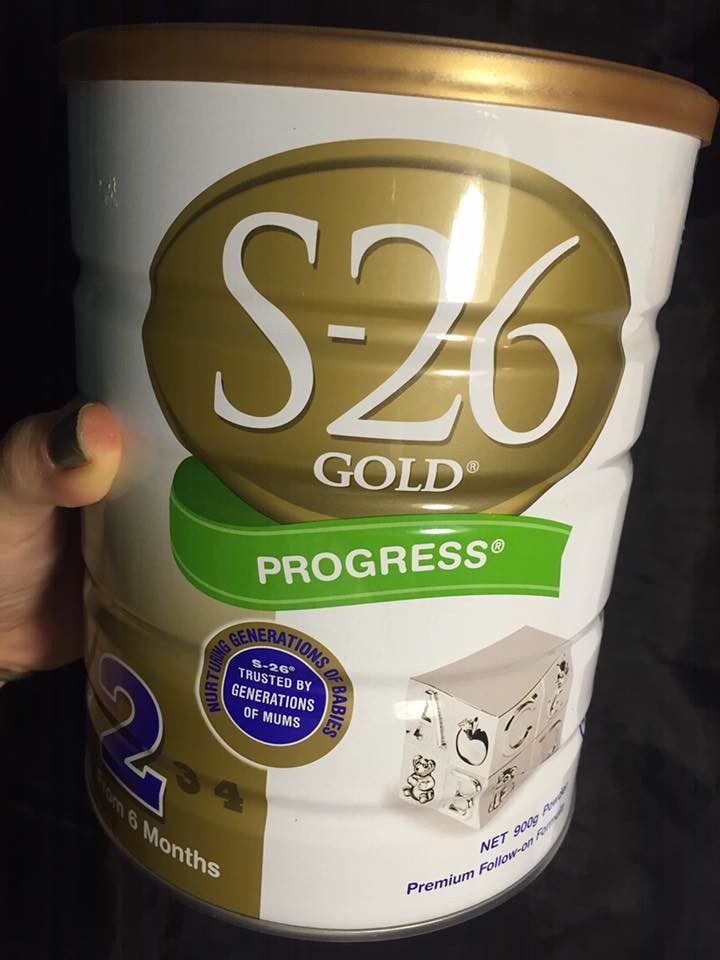The photograph depicts a person holding a white metal canister with a gold plastic snap-on lid. The background is a uniform dark, possibly black sheet, adding contrast to the scene. The person’s thumb, adorned with dark fingernail polish, is visible as they grasp the canister. The canister features prominent gold and green accents. At the center top, a gold oval with white text reads "S-26 Gold". Below this, a green banner with white text states "Progress". Further down, a gold banner says, "Nurturing Generations of Babies S-26 Trusted by Generations of Moms". A bright blue "2" appears on the left, with a gray "3" and "4" next to it. On the bottom right, the text "From 6 Months Premium Follow-On Formula" is displayed. An additional detail includes a silver block with an apple and a bear in black and white on it, indicating letters associated with these images. The overall composition highlights both the product details and the contextual environment.